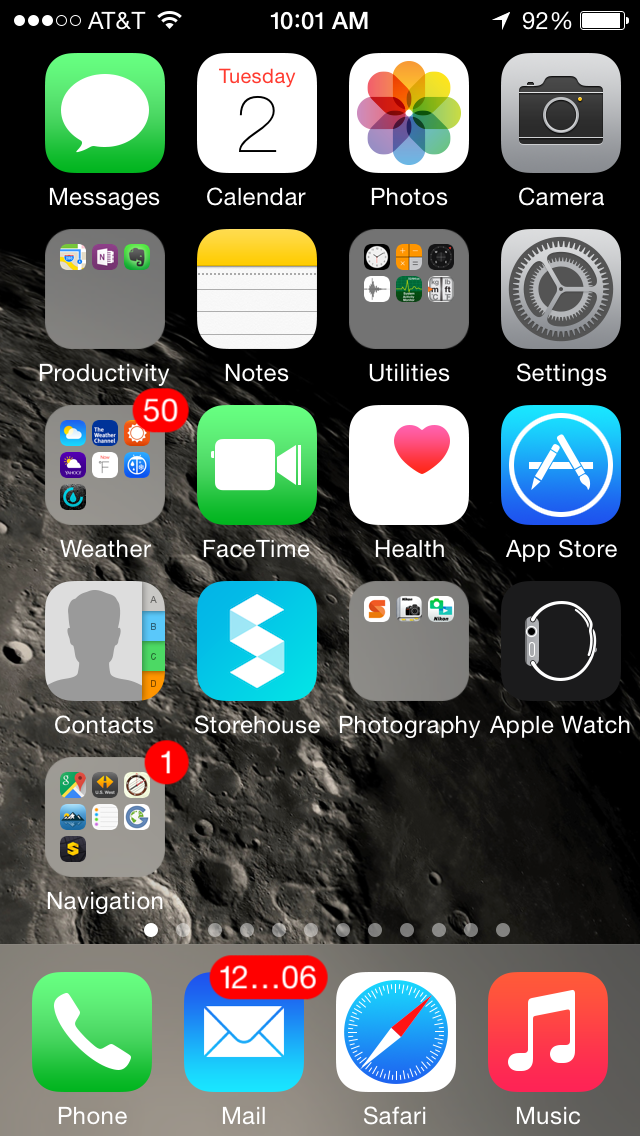This is a detailed screenshot of an iPhone home screen. The screenshot clearly shows characteristics that identify it as an iPhone, such as the distinct top status bar layout and icons arrangement. 

At the very top, there are three solid white circles alongside two clear ones, which indicate signal strength. To the left of these, a small banner displays "AT&T," next to the Wi-Fi indicator. In the center, the time is clearly shown as 10:01 a.m. Toward the right, an arrow points to "92%" next to a mostly full battery icon, which has a very thin border at the top.

The background of the screen is a dark, zoomed-in image of the moon, capturing detailed craters and surface textures. Arranged over this background are various app icons. From left to right, top to bottom, some identifiable apps include Messages, Calendar, Photos, Camera, the App Store, and an Apple Watch section.

Additionally, there are folders containing multiple apps for better organization, such as a photography folder and a navigation folder. These folders have small icon grids inside them indicating they contain several apps. 

At the bottom center of the screen, a series of small circles, eight in total, signifies that there are multiple pages of apps available, with the first circle filled to indicate the current page.

Below these circles, a gray banner holds four primary app icons: Phone, Mail, Safari, and Music. The Mail icon specifically indicates a high volume of new messages with a red notification badge displaying "1206."

This comprehensive layout provides a clear and detailed look at the user's iPhone home screen, capturing both the static elements and dynamic notifications effectively.